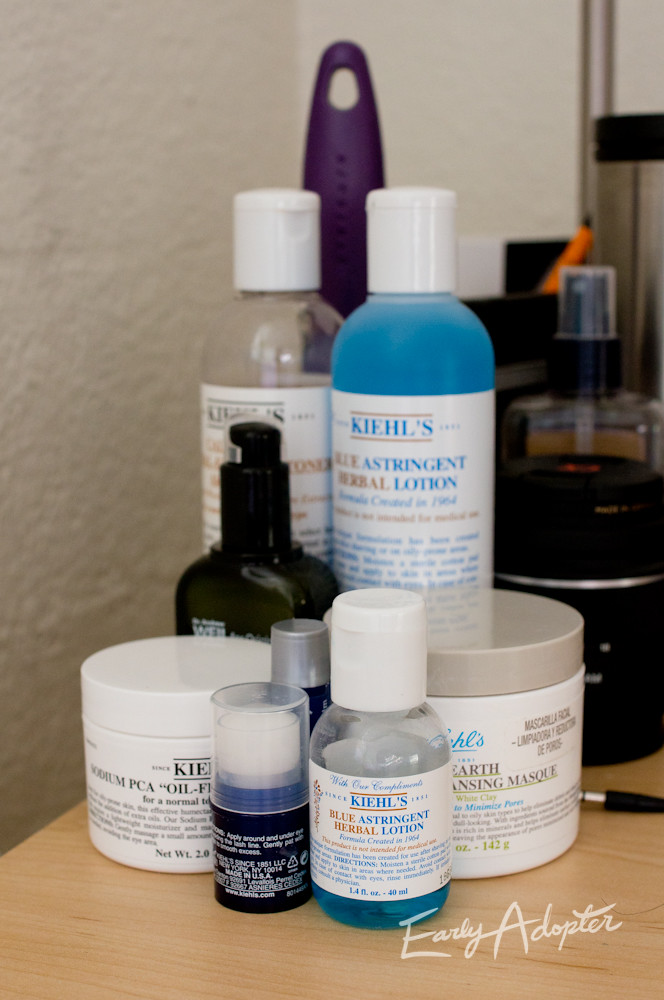In this image, there are eight distinct products displayed, which appear to be a variety of personal care items, likely focused on hair care. The arrangement includes two larger bottles, three smaller bottles, and two container-like products. The labels on these items mostly read "Kiehl's," indicating the brand. 

To the back, there are two similarly sized bottles: one is fully filled with a blue substance and labeled "Herbal Lotion," while the adjacent bottle seems to be the same kind but is empty. Between these larger bottles, there is a smaller bottle that has a dark black or very dark green color. Among the containers, one label clearly states "mask," suggesting the presence of a hair mask or facial mask product. Three more small bottles are centrally placed between the two container-like products.

Overall, the collection is grouped together on a table, giving the impression of a cohesive set of hair care or lotion products. At the bottom, there is a printed phrase "early adopter," hinting at a promotional or new product release.